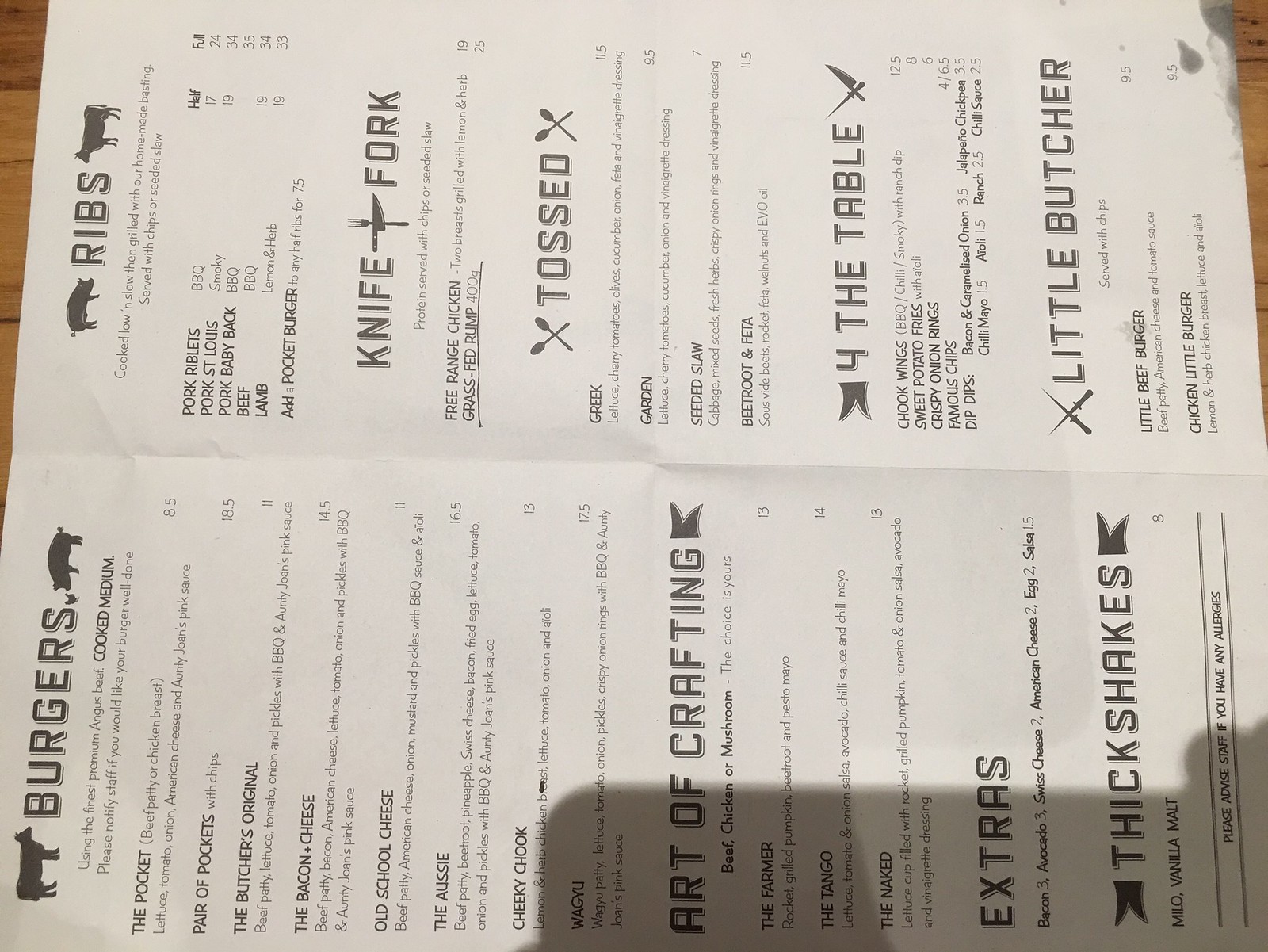This photograph showcases the interior menu of a restaurant, albeit taken sideways, making it more difficult to read. The menu is printed on thick, white paper with black text set against a clean white background. The menu is organized into several categories: Burgers, the Art of Crafting, Extras, Thick Shakes, Ribs, Knife and Fork, Tossed for the Table, and Little Butcher. 

Under the Burgers section, options include the Old-School Cheeseburger, Bacon Cheese, and the Butcher's Original. The menu also offers a variety of salads such as Greek Salad and Garden Salad. The Ribs category features selections like Pork Riblets, Beef Ribs, Lamb Ribs, and Pork Baby Back Ribs. The "For the Table" section appears to cater to group dining, featuring shareable items like wings and onion rings. The Little Butcher section likely contains kid-friendly or smaller portioned meals. The menu’s extensive variety appears inviting, catering to a wide range of tastes and preferences.